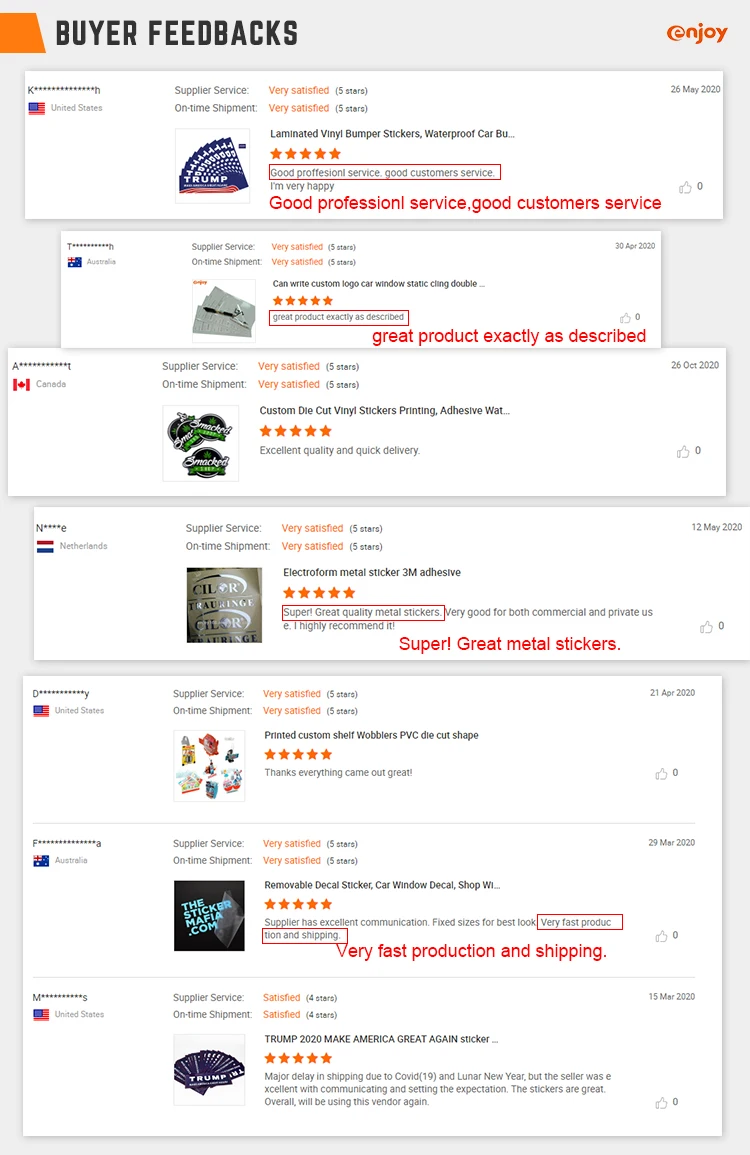The display presented showcases the "Buyer Feedbacks" section from Enjoy. The title "Buyer Feedbacks" is prominently displayed in black font, accented by a vertical orange stripe on the left side. The term "Enjoy" is written in a distinctive format, with a lowercase "e" stylishly wrapped in orange, followed by "njoy" in the same vibrant hue. 

The layout is visually impressive, but some text becomes unclear upon zooming. The display features an image of laminated vinyl bumpers along with excerpts from various customer testimonials. Key remarks include:
- "Good professional service, good customer service."
- Ratings with comments such as "Great product, exactly as described," "Super great metal stickers," and "Very fast production and shipping."

Visible product descriptions encompass:
- Custom die-cut vinyl stickers.
- Printing services.
- Printed custom sheer materials.
- A controversial sticker reading "Trump 2020 Make America Great Again," which elicited a negative reaction.

Overall, this feedback section illustrates Enjoy's diverse offerings and highlights both customer satisfaction and occasional polarizing content.